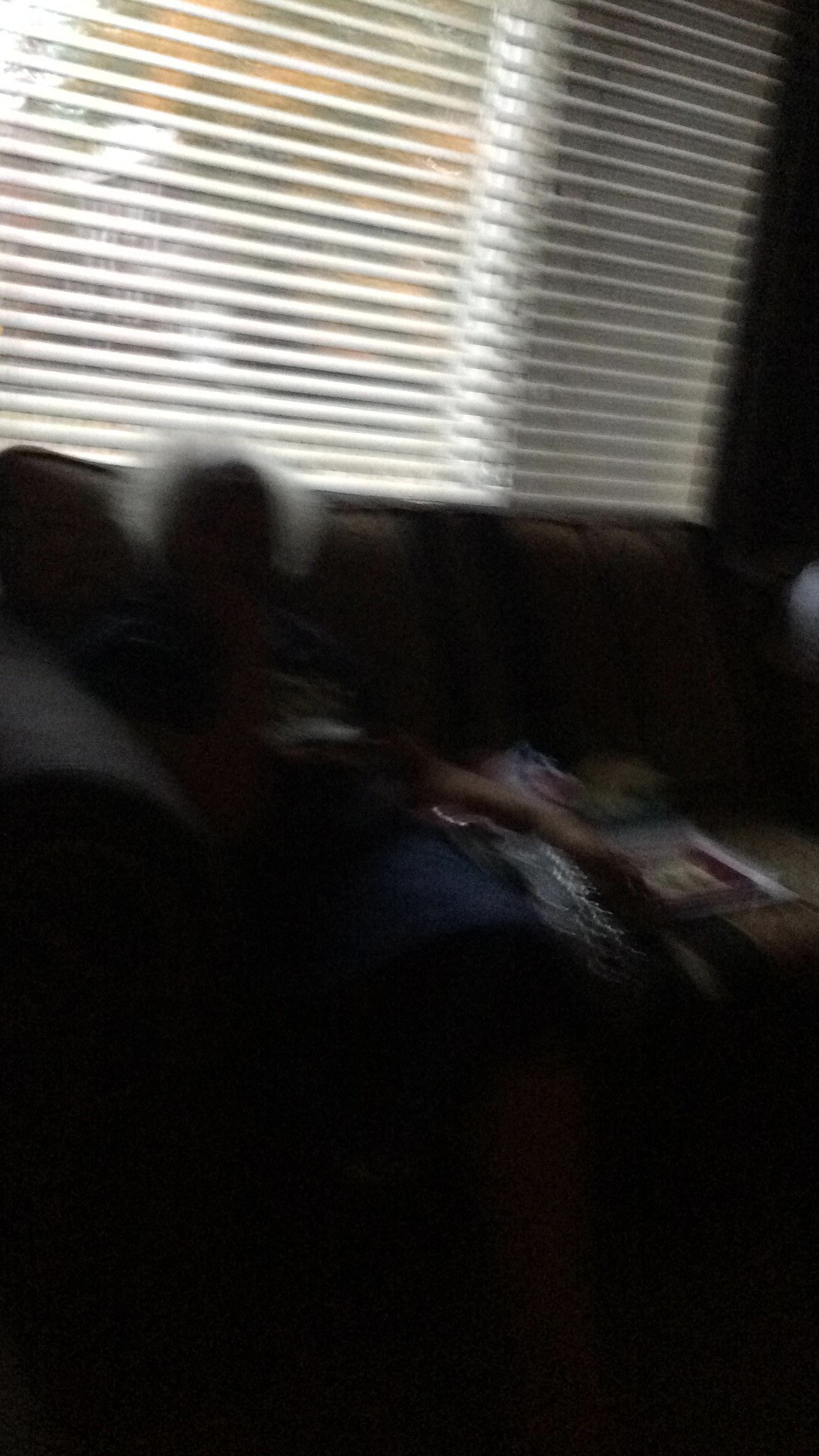The image is a tall, narrow photograph that is roughly two and a half times taller than it is wide. It is incredibly blurry and dark, with the bottom third of the frame pitch black and indiscernible. The upper part of the image features a window adorned with white Venetian blinds that are halfway open, allowing some sunlight to filter into the room. Outside the window, there is foliage with shades of green and yellow, suggesting either an autumnal scene or spring blossoms. Distant, out-of-focus background buildings, white and brick, can also be seen.

Directly below the window is a dark brown couch, barely visible in the low light. On the far left side of the couch, there is an indistinct figure seated. The person appears to be an elderly individual, characterized by frizzy gray hair silhouetted against the dark background. Their silhouette suggests that they are sitting up, possibly with a blanket covering them, revealed by faint shades of blue and red halfway down the image. Their right arm is raised towards their face, and their left arm rests on the couch. Next to them on the couch, there is a cluster of blurry objects in various colors, possibly including a red and green blanket and a silver item. These contributions to the overall scene add complexity to the dimly lit, tranquil setting.